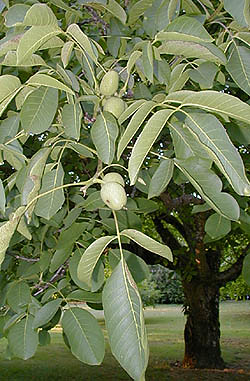The photograph, somewhat faded, captures a vibrant outdoor scene during daytime in a lush nature area. The primary focus of the image is an imposing, ancient tree, its thick trunk situated on the right-hand side of the frame. Surrounded by a rich, green open field, this solitary tree stands out as a testament to nature's splendor. The trunk rises approximately four feet before giving way to numerous robust branches. These branches reach out and up, supporting an abundance of large, vibrant green leaves, characterized by their ash-like shape, although the tree itself is not an ash. Amidst the greenery, clusters of green, grape-like fruits can be seen, possibly mangoes, though they are not yet ripe. These fruits, numbering three or four, add a touch of potential future bounty to the scene. The overall impression is one of an old, majestic tree thriving in a verdant, grassy expanse, exuding an air of health and vitality.